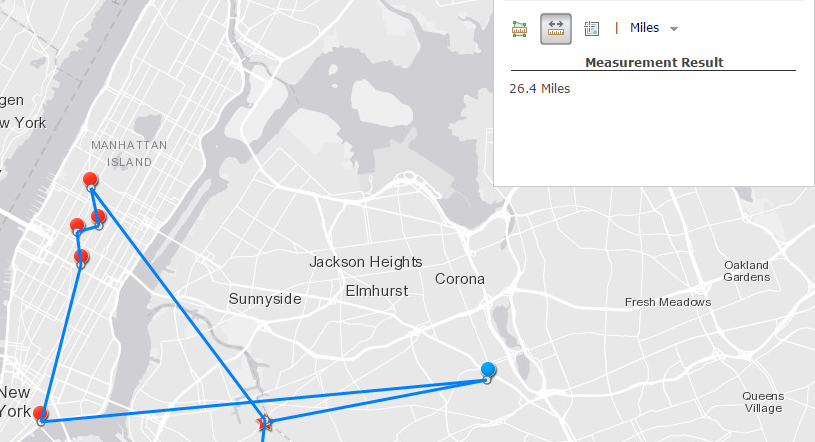This is a detailed photograph of a map accompanied by a legend. The map, predominantly rendered in shades of gray and white, evidently depicts Manhattan Island along with portions of Long Island and possibly Staten Island. Points of interest are marked by red dots that feature a white edge, while royal blue lines connect these points. Notably, a red star marks a significant location through which these blue lines pass. Additionally, a singular blue dot with a white edge is also visible. Prominent text on the map includes place names such as Manhattan Island, New York; Sunnyside; Jackson Heights; Elmhurst; Corona; Fresh Meadows; Oakland Gardens; and Queens Village. The accompanying legend, titled "Measurement Results," indicates a total distance of 26.4 miles, which the blue lines appear to chart. At the top, the word "Miles" is present with a dropdown menu beneath it.